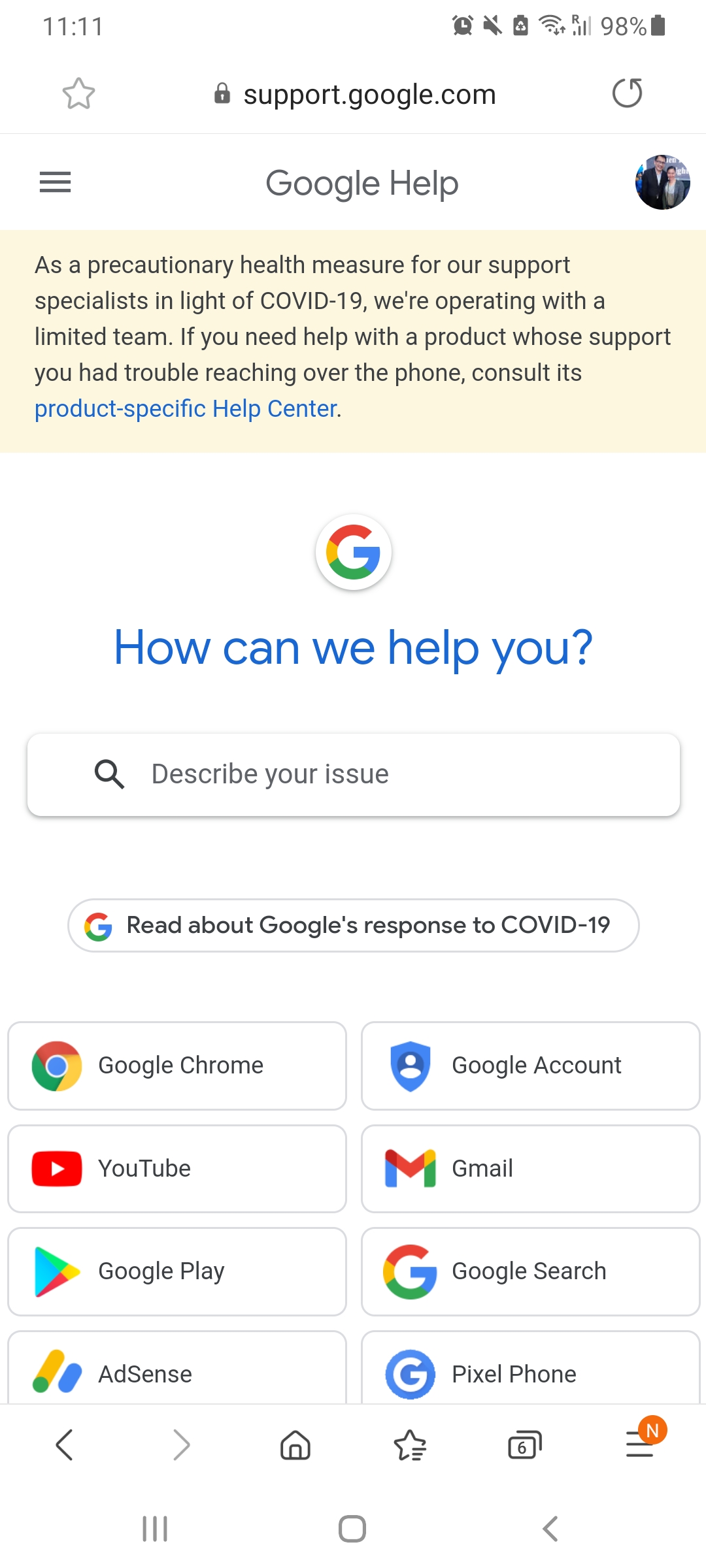**Detailed Descriptive Caption:**

The image is a screenshot taken on a mobile phone, displaying the support.google.com webpage at 11:11 AM. At the top, there is a notice addressing the impact of COVID-19 on Google's support services. The message informs users that due to precautionary health measures for their support specialists, Google is operating with a limited team. Users experiencing difficulty reaching product support via phone are advised to consult the product-specific help center.

Below the notice, the Google 'G' logo is prominently featured, followed by a query prompt, "How can we help you?" A rectangular search box with a magnifying glass icon invites users to describe their issues. Beneath the search box, a horizontal bubble directs users to "read about Google’s response to COVID-19."

Further down, a series of tabs categorizing various Google services are displayed. These include: 
- Google Chrome
- Google Account
- YouTube
- Gmail
- Google Play
- Google Search
- AdSense
- Pixel Phone

Each tab is accompanied by its respective logo. At the bottom of the screen, standard mobile navigation icons are visible, including the back button, forward button, and a home star for favoriting items, alongside an indication of the number of open tabs and other typical phone control buttons.